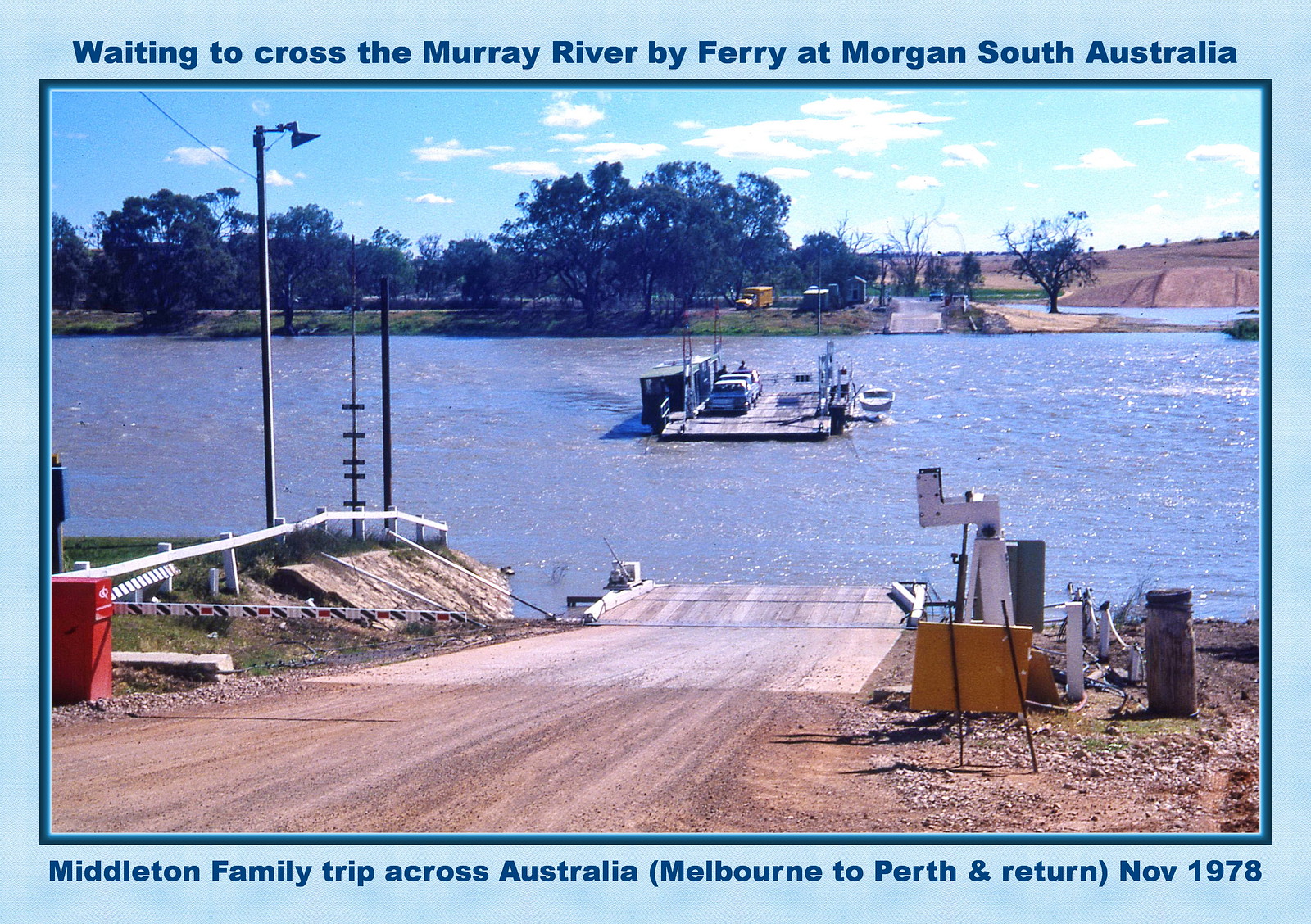The image showcases a photograph bordered by a light blue digital frame with dark blue text at the top and bottom. The top text reads, "waiting to cross the Murray River by ferry at Morgan, South Australia," while the bottom text states, "Middleton family trip across Australia, Melbourne to Perth and return, November 1978." The photograph is enclosed within a dark blue sub-frame. 

Within the image, a boat ramp starts from the bottom left and extends towards the center, where it meets a waterway running horizontally across the middle of the image. The ramp is bordered by a white fence on the left and streetlights mounted on lamp posts. The dirt path to the ramp is brown, and various signs face the river on the right side of the path.

On the water, a small ferry boat carries a few cars and a rescue raft attached to its side. In the background, the opposite shoreline features grassy areas and trees, especially toward the left, with additional ramp access on the right. The distant shore also shows small mounds of dirt and more trees. The sky is a brilliant blue with scattered white clouds, indicating a sunny day.